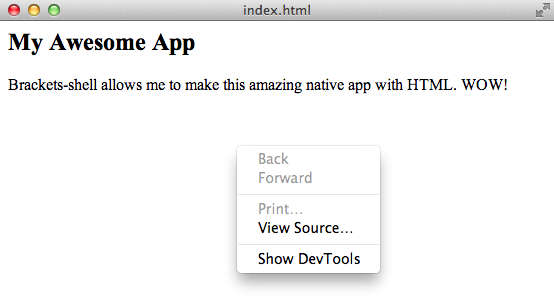A detailed caption describing the screenshot of a web test page:

"The screenshot captures a test page with a clean, white background. At the top, a gray bar features three circles in the top left corner - red, yellow, and green, reminiscent of browser window controls. To the right of these circles, 'index 8.html' is displayed alongside two small diagonal arrows pointing right and down, indicating options to expand. Below the bar, the text reads, 'My awesome app – shell allows me to make this amazing native app with HTML. Wow!' Additionally, a context menu is visible, showing options: 'Back,' 'Forward,' 'Print' (all grayed out), 'View Source,' and 'Show Dev Tools,' suggesting the menu was activated by a right-click action on the page."